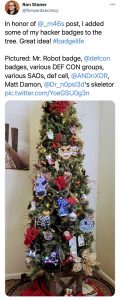In this low-resolution image, we see a Christmas tree adorned with a myriad of unique ornaments, positioned in the corner of a room with white walls. There's a picture hanging on the wall behind the tree, though its details are unclear due to the blurriness. The tree itself is lush and green, festooned with diverse ornaments of various colors, sizes, and designs, including faces.

The image appears to be a social media post, likely from Twitter, although the details are somewhat difficult to decipher. The post mentions that in honor of a user (@_m46s), the poster added several hacker-themed badges to the tree. The caption reads: "In honor of @_m46s post, I added some of my hacker badges to the tree. Great idea! #badgelife," and lists several specific badges: Mr. Robot badge, DefCon groups, SAOs from DefCell, @andxor, Matt Damon, @dr_n0pes, psi3d, and Skeletor. The tweet includes a link to a picture (pic.twitter.com/...).

Despite the blurriness, the creativity and homage to hacker culture are evident in the detailed and distinctive decorations on the Christmas tree.